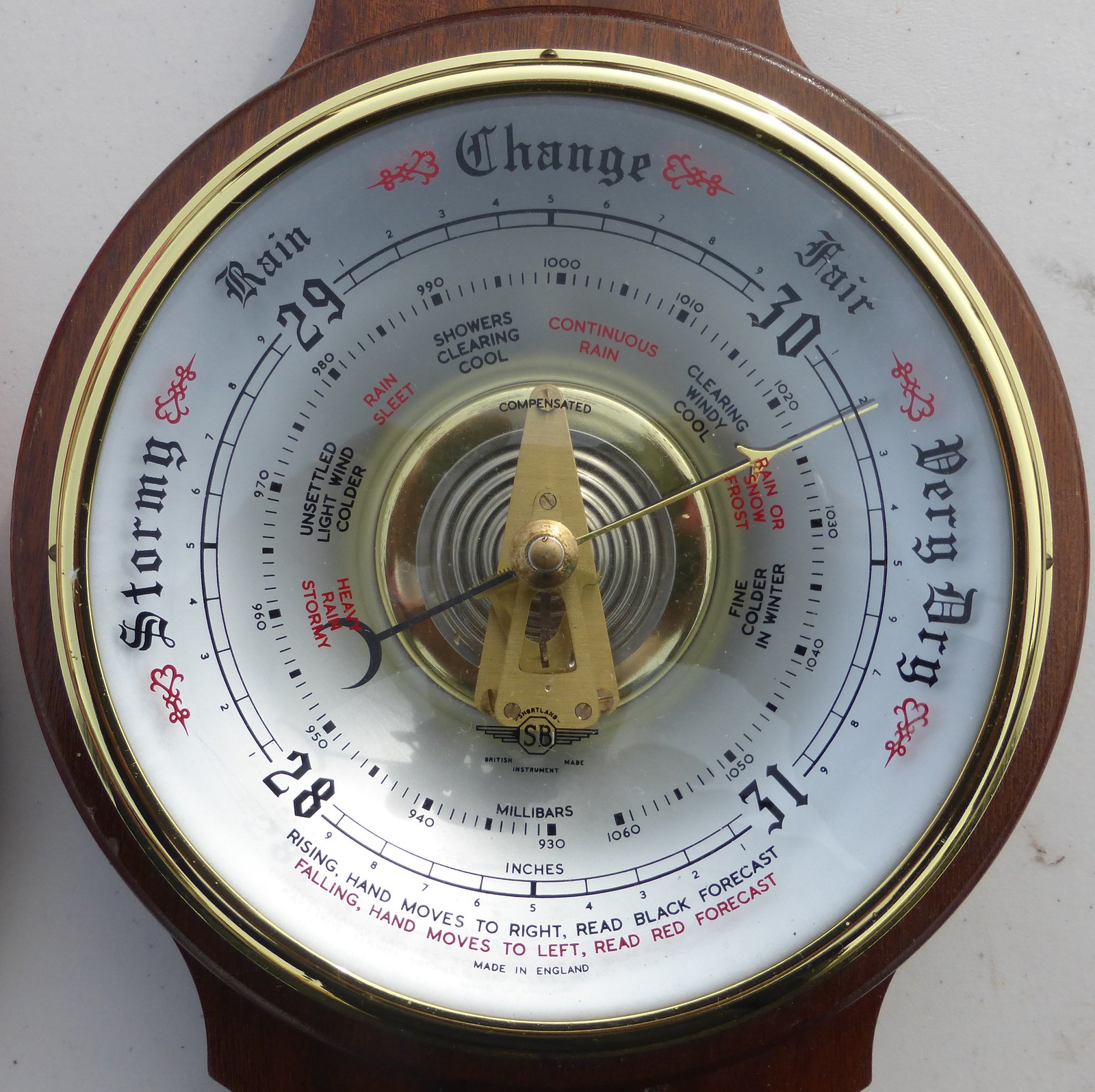The image is a detailed close-up photograph of a barometer, designed to predict the weather. The device prominently features a golden dial with a brown wooden border. Around the outer edge of the dial, key weather conditions are marked: "stormy," "rain," "change," "fair," and "very dry." The barometer dial includes numbers ranging from 28 to 31 to indicate atmospheric pressure, with smaller units perhaps in millibars.

The device has a central hand resembling a clock's, with an arrow on one side and a crescent shape on the other. Various weather descriptors circle within the outer ring, including "heavy rain," "stormy," "unsettled," "light wind," "colder," "sleet," "showers," "clearing," "cool," and "rain or snow," with notes for "continous rain," "windy," "cool," "frost," and "fine, colder in winter." 

At the bottom of the dial, instructions indicate the barometer's usage: "Rising hand moves to right, read black forecast. Falling hand moves to left, read red forecast." Below this, in smaller text, it reads "Made in England." Overall, this barometer combines functional precision with aesthetic detail capturing various weather conditions and pressure measurements.